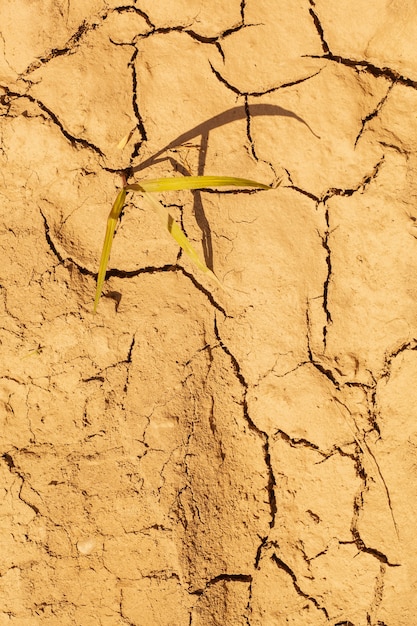This vertically oriented rectangular photograph captures a close-up view of an extremely dry, cracked ground resembling a parched riverbed or desert landscape. The light tan to golden brown soil is riddled with a network of wide and narrow crevices, which appear almost black due to the sharply defined shadows cast by the bright sunlight. Adding a touch of life to the arid scene, a small plant with three elongated, narrow, pointy leaves—pale greenish-yellow in color with a hint of brown at the ends—emerges from the dirt. The plant's leaves, along with a thin brown stem, cast distinct, clearly defined shadows on the parched earth beneath them.